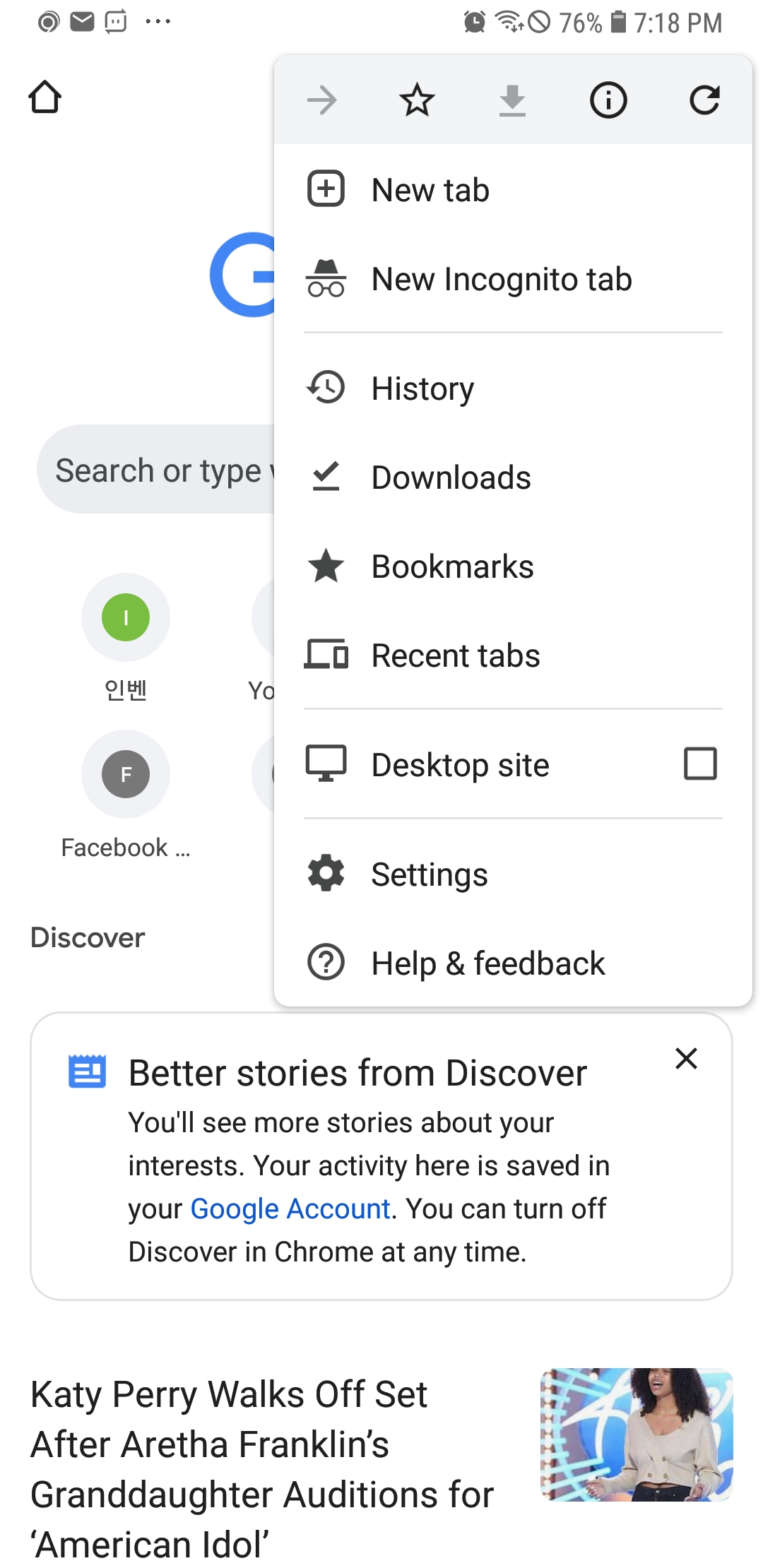### Detailed Caption:

A detailed screenshot of a smartphone displaying a search page on Google Chrome. At the top left of the screen, "Email" is visible, indicating the source of the app notification. The status bar shows an alarm icon, Wi-Fi signal strength, current battery percentage at 76%, and the time as 7:18 PM. Below the status bar, the browser's interface includes options such as "New tab," "New incognito tab," "History," "Downloads," "Bookmarks," "Recent tabs," "Desktop site," "Settings," and "Help and feedback."

The main content of the screen is under the Google search and address bar, which has a “G” logo and a house icon on the left side. It features a Discover card showcasing a headline: "Katy Perry walks off set after Aretha Franklin's granddaughter auditions for American Idol." Below this, there's content in Chinese characters, and suggestions about Facebook along with an explanatory note about Discover’s functionality: "Discover better stories from Discover. You'll see more stories about your interests. Your activity here is saved in your Google account. You can turn off Discover in Chrome at any time."

In the bottom-right corner, there is a rounded-icon image of a monkey dressed in a shirt against a blue circular background with white text. However, upon closer inspection, it is mentioned as being a person in a monkey costume, contributing to a somewhat humorous or whimsical element in the otherwise technical and informational screenshot.

(Note: The inappropriate language used in the original description has been omitted to maintain a respectful and professional tone.)